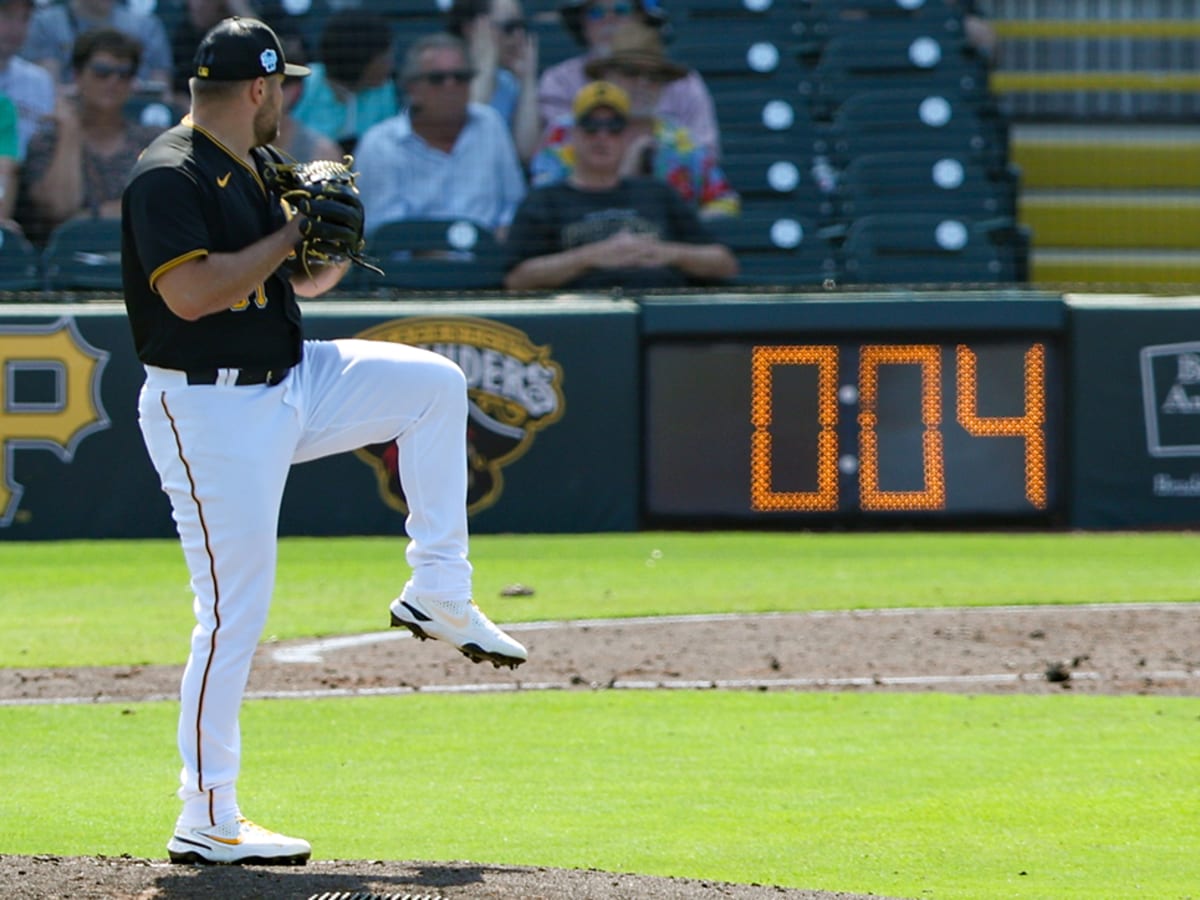A high-detail photograph taken during a baseball game captures a pivotal moment as a pitcher, clad in a black Nike jersey and matching black cap, with white pants, prepares to throw the ball. The player stands on the left side of the image, one leg raised and both hands securely placed in his black glove. He also wears white baseball cleats. The background features a digital timer that reads '0-0-4,' indicating that there are four seconds left on the clock. The well-maintained field, with its light green grass, and the crowd seated in the stands, many of whom are wearing sunglasses, can be slightly observed, though they remain somewhat blurred. A yellow 'P' is noticeable at the bottom of the stadium, and an unreadable team sign also adorns the background, hinting at the lively and sunny ambiance of the game day.